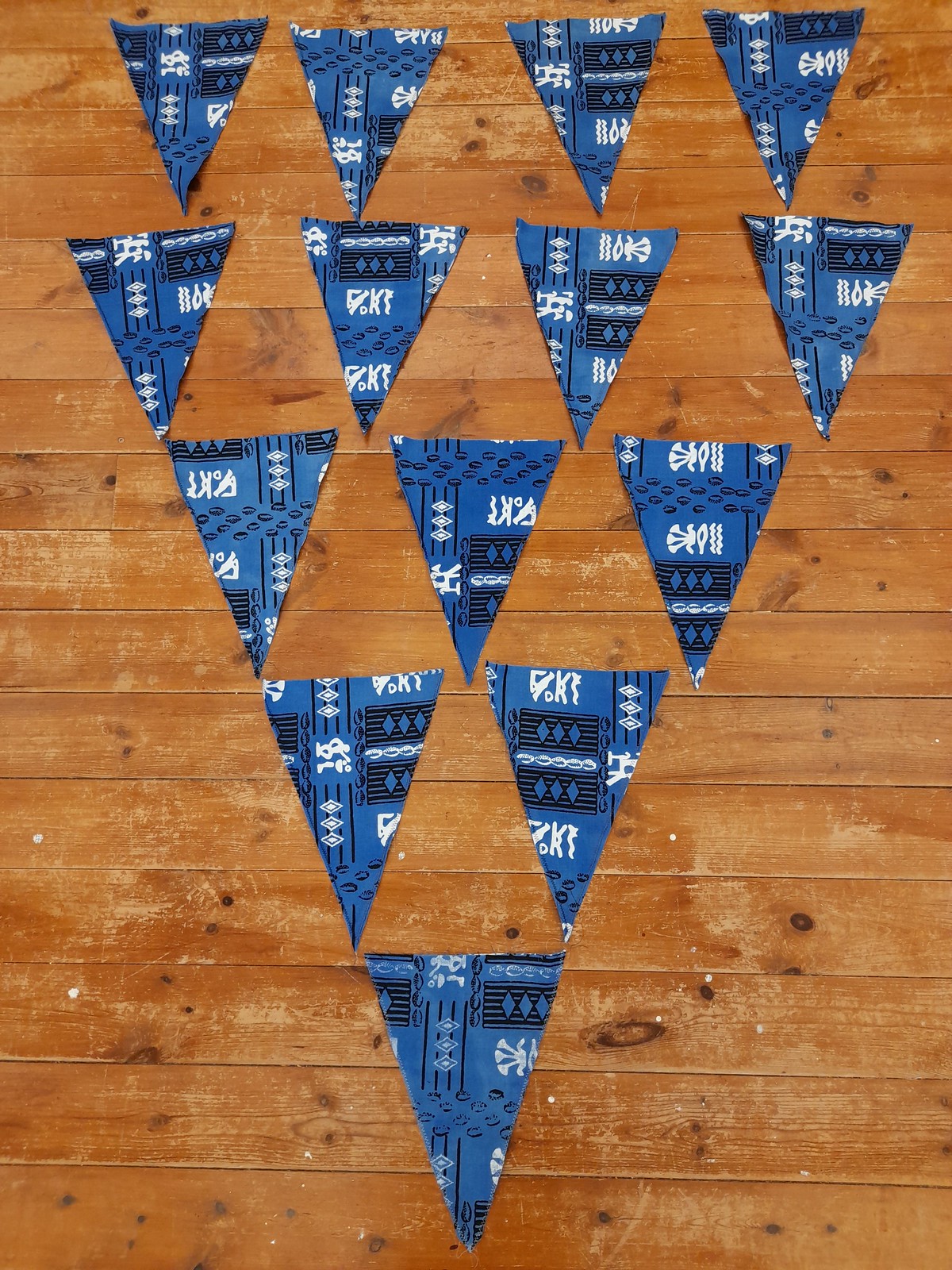This is a detailed photograph of 14 blue fabric triangles arranged in a larger triangular formation on a worn light-brown wooden surface. The rows of triangles consist of one at the bottom, two above that, three above that, and two rows of four at the top. The wood appears weathered, with horizontal narrow planks featuring visible knots, grain, and scratches. Some steel nails can be seen on the far left. The fabric triangles have a blue base adorned with black stripes and abstract black and white designs, with each triangle showcasing a different section of the fabric. The material of the triangles resembles cotton bandana fabric, adding a tactile element to the visual composition. Photographed at an angle, the bottom triangle appears larger and closer, while the top ones diminish in size and distance, enhancing the depth of the image.